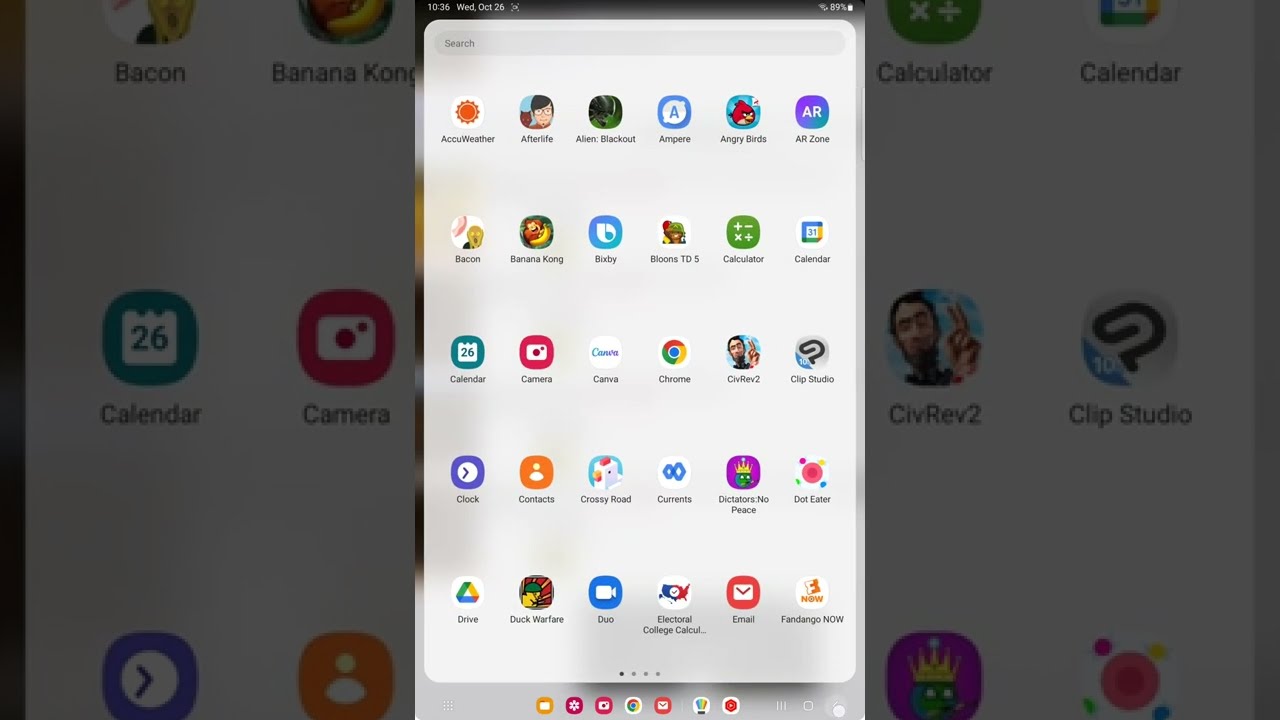The image is a detailed screenshot of a tablet’s home screen and app tray. At the center, there is a vertically oriented rectangular app tray with a white background, displaying 30 app icons in a structured grid of six columns and five rows. The upper left-hand corner of the tray features the AccuWeather icon, marked by an orange sun. Adjacent to this is the Afterlife app icon, depicting a young boy with black hair and glasses, followed by the Alien Blackout icon with an alien image. Below these icons are various other familiar app icons like Angry Birds, Civilization II, Clip Studio, Google Drive, calculator, calendar, and camera. The background of the image is darker and somewhat faded, offering a stark contrast to the central app tray. Additionally, there's a taskbar at the bottom of the screen, highlighting selected options such as settings, Google Chrome, and email. Just above the taskbar are four circles, the first being black and the subsequent three lighter gray, indicating possible navigation through multiple pages within the app tray. The overall background, while light and slightly transparent, primarily accentuates the central app tray and its contents.